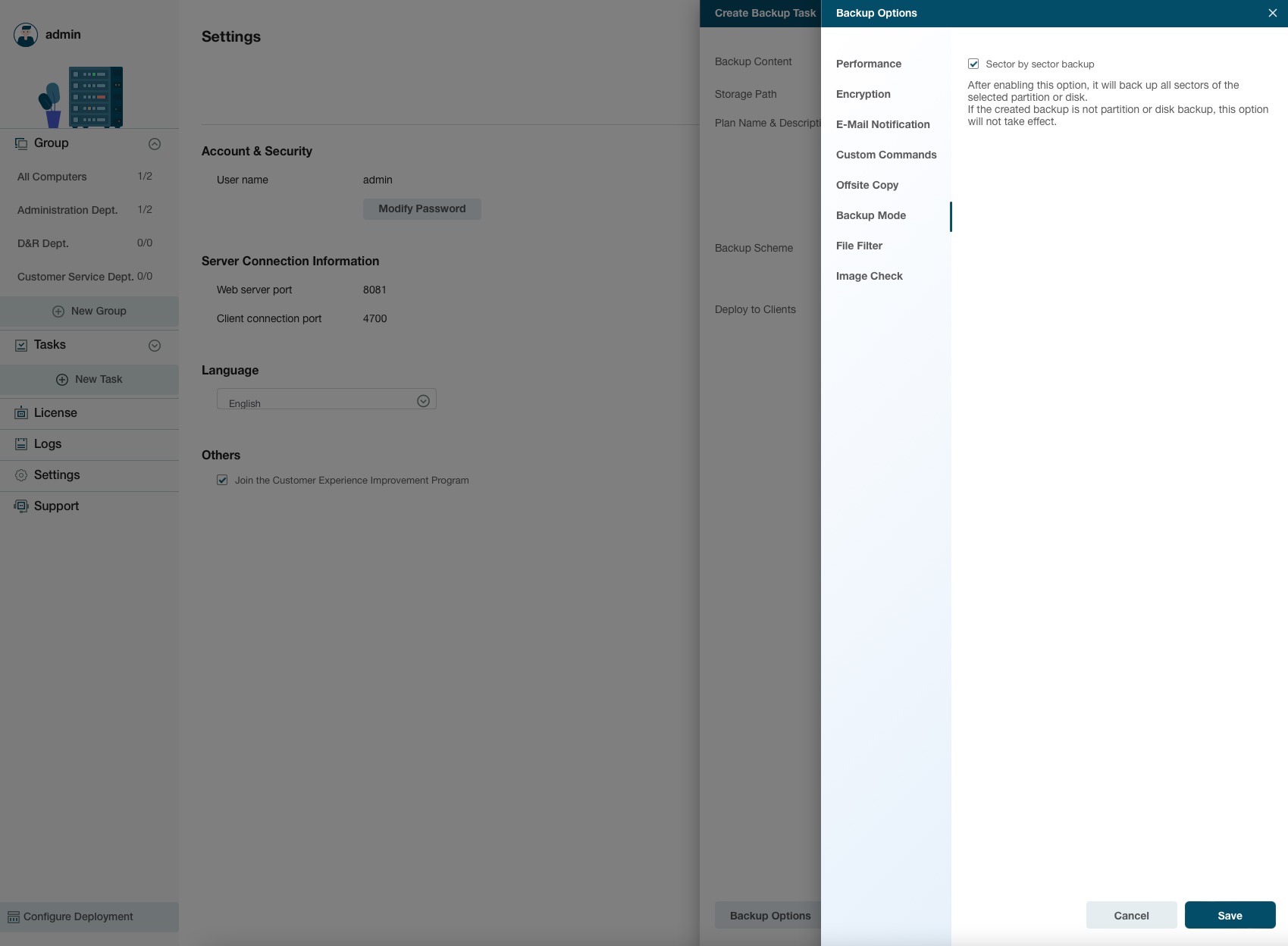The image depicts a computer screen where a user is configuring their backup options. The screen is primarily divided into two sections. The left two-thirds is shaded gray, representing the administrator settings for the computer, while the right third is a focused, white pane where backup options are being set.

In the right section, the white pane is topped by a blue bar with the text "Backup Options" in white. Directly below, the pane lists various backup configuration choices in a vertical column on the left: Performance, Encryption, Email Notification, Custom Commands, Off-Site Copy, Backup Mode, File Filter, and Image Check. On the right side of this pane, there is a checkbox labeled "Sector by Sector Backup" with a blue check mark. Beneath this, a gray text explains the function: "After enabling this option, it will back up all sectors of the selected partition or disk. If the created backup is not partition or disk backup, this option will not take effect."

At the bottom of the white pane are two buttons: a gray "Cancel" button on the left and a dark blue "Save" button on the right, both with corresponding text.

The administrator settings on the left, which are grayed out, include an icon and the word "Admin" at the top left, followed by various setting options: Settings, Account Security, Username (admin), Modify Password, Server Connection Information, Web Server Port (8081), Client Connection Port (4700), Language (English via a drop-down box), and a checkbox for "Join the customer experience improvement program." Additional administrative options include Group (with sub-options like All Computers, Administration Department, DNR Department, Customer Service Department, New Group), Tasks, New Task, License, Logs, Setting, and Support.